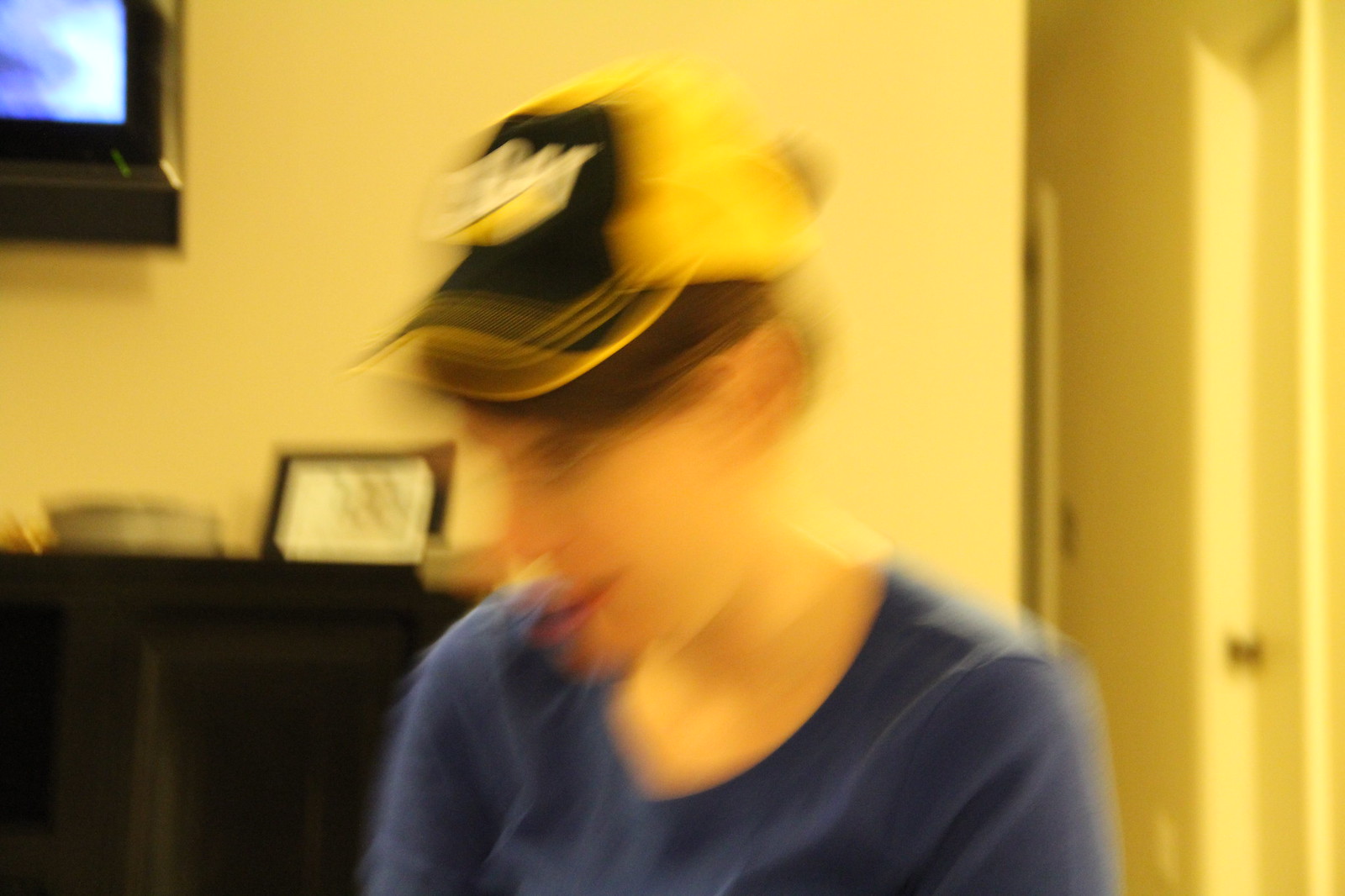This is a blurry indoor photograph that captures a person standing in what appears to be a living room leading to a hallway. The individual wears a blue shirt and has brown hair, which is tucked up in a yellow and black cap that bears the "CAT" logo, commonly associated with construction brands. While the person's gender is not entirely clear, the overall presentation suggests they might be female, despite the more masculine appearance of the hat. The walls of the room are painted white, and the ambient lighting imbues the scene with a subtle yellowish glow. To the left of the person, there is a piece of black wooden furniture adorned with a picture frame and various other small objects.